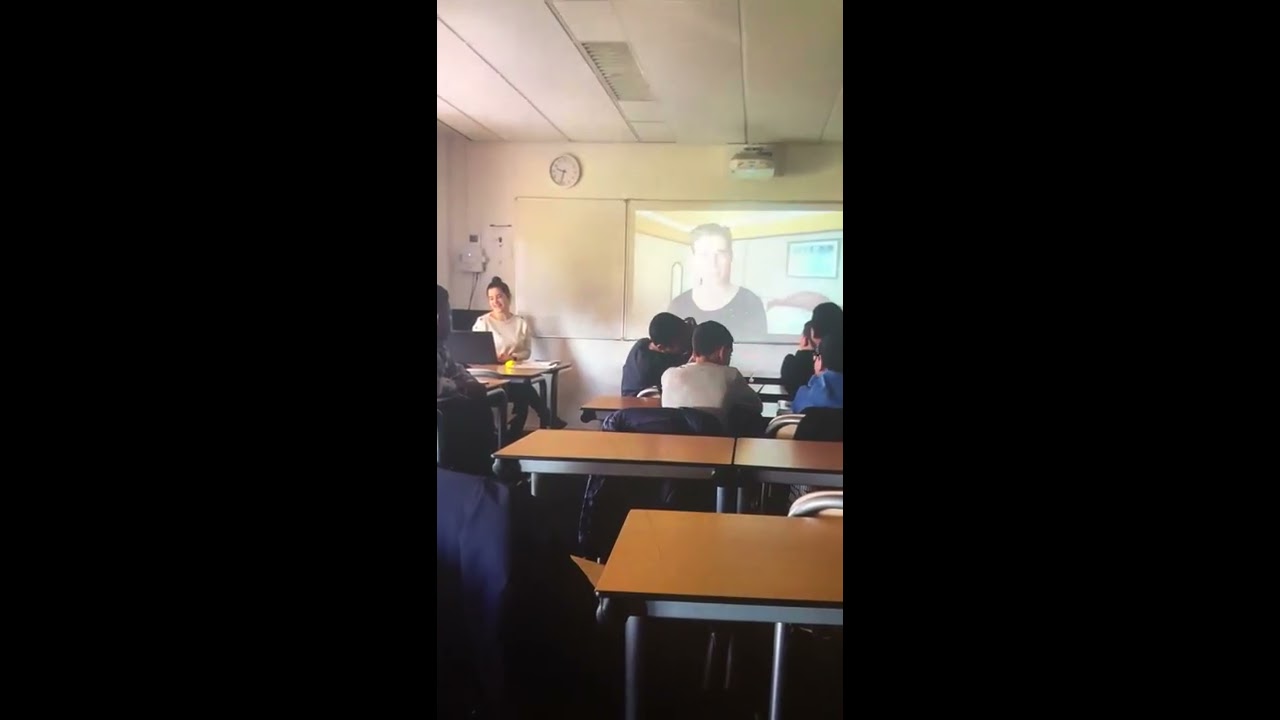This photograph captures a classroom scene from the back, focusing on three empty desks at the forefront. The students, more visible toward the right side, are seated at long brown tables with gray bases and tan chairs. A central feature is a video projection on the white wall at the front of the room, indicating a possible class activity. The lighting in the room suggests it is daytime, with white walls and ceiling contributing to the brightness filtering through. A clock on the upper left wall shows 9:30, situating us in a specific moment of class time. Below the clock, the instructor's desk is visible, where a woman in a white shirt and dark pants sits facing the students, engaging with her open laptop. The students' attire varies from a darker blue shirt, a white or tan shirt, to a blue hoodie, with another individual in dark clothing. Thick, black vertical lines frame the image on both sides, possibly due to the image's format.